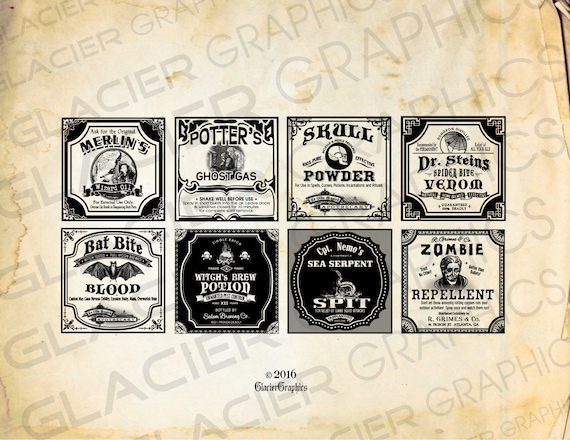The image displays a grid of eight distinctive stamps arranged in a four-by-two layout, each representing fictitious businesses with a macabre theme. The background resembles an old, parchment-like scroll with a tan, beige hue and is subtly overlaid with a translucent watermark that says “Glacier” repeatedly, giving it a vintage vibe. Each stamp contains unique graphics and text:

1. **Top Row, First Stamp**: "Merlin's Wizard Oil" features a circular illustration possibly depicting a wizard.
2. **Top Row, Second Stamp**: "Potter's Ghost Gas" shows a ghost hovering over a seated figure.
3. **Top Row, Third Stamp**: "Skull Powder" presents a black circle with a white skull at its center.
4. **Top Row, Fourth Stamp**: "Dr. Stein's Spider Bite Venom" includes a circular image of a spider web.

5. **Bottom Row, First Stamp**: "Bat Bite Blood" displays an illustration of a black bat.
6. **Bottom Row, Second Stamp**: "Witch's Brew Potion" has a predominantly black background with white text.
7. **Bottom Row, Third Stamp**: "Captain Nemo's Sea Serpent Spit" is set against a grey background with a black circle, featuring white text.
8. **Bottom Row, Fourth Stamp**: "Zombie Repellent" highlights a zombie's head between the words, with a white box and a black dotted border.

Additionally, there is a copyright notice at the bottom that reads “© 2016 Glacier Graphics.” Each stamp is meticulously designed to reflect its eerie theme, enhancing the overall spooky aesthetic of the image.